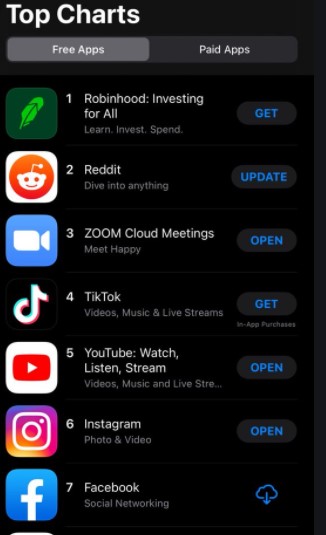A screenshot from a cell phone app store showcasing the "Top Charts" section against a black background. In the upper left corner, the title "Top Charts" is displayed in white text. Below it, two rectangular labels appear: "Free Apps" on a gray rectangle and "Paid Apps" on a darker gray rectangle to the right.

The list begins on the left with an icon of a green leaf in a square, adjacent to the text "Robinhood: Investing For All." To the right, there is a blue button labeled "Get." 

Next, "Reddit" is listed at number two with an "Update" option beside it. Following this, "Zoom Cloud Meetings" occupies the third position, featuring a blue square with a video camera icon and an "Open" button to the right.

"TikTok" ranks fourth with a "Get" button on its right side. "YouTube: Watch, Stream, Listen" is fifth, showcasing a red box with a white play arrow and the "Open" option. 

Subsequently, "Instagram" is listed, its rainbow gradient icon (pink, yellow, and purple) leading to an "Open" button in blue.

Finally, "Facebook" ranks seventh, displayed with a blue square featuring a white lowercase "f" alongside a cloud icon with a downward arrow for updating the app. This label marks it as part of the Social Networking category.